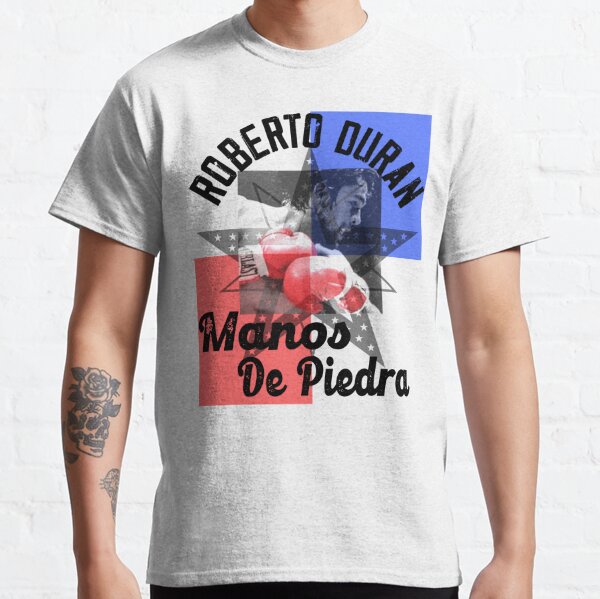The photograph showcases a model wearing a white short-sleeved t-shirt, posed against an almost indistinguishable white brick wall. The shirt features black text that reads "Roberto Duran" in a semi-circular formation at the top and "Manos de Piedra" at the bottom, framing a slightly faded image of a boxer with red Everlast gloves. Between these phrases, the image of the intense boxer, viewed from the side, is set within a black square, with a red square at the bottom left corner. Additionally, superimposed over the boxer is a five-pointed star filled with smaller stars. The model's head and everything below the shirt are cropped out, emphasizing the shirt's design. The model also has a distinctive skull and rose tattoo on his right arm, adding a striking element to the composition. The t-shirt's color appears white but might have slight grayish or light blue tones.